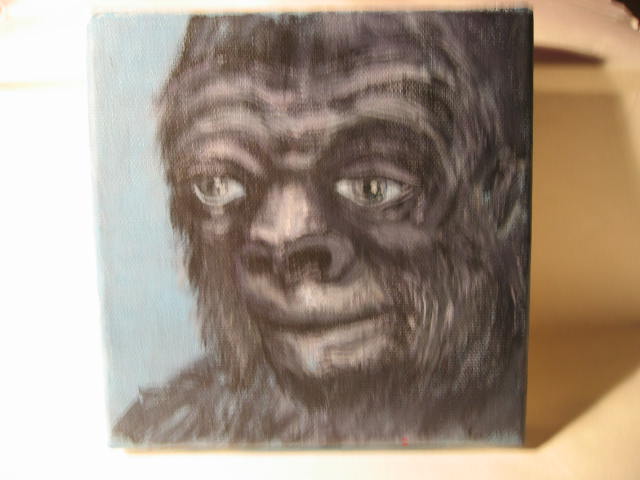The image displays a photograph of a canvas painting. The canvas, standing upright, features a detailed close-up of a primate-like creature with a blank expression and black fur. Its eyes are light grey and have a very human-like appearance, contributing to the creature's neutral demeanor. The composition captures the creature from the collarbone up, focusing on its large snout and partially concealed mouth. The background of the painting is light blue, providing a stark contrast to the creature's dark fur.

The canvas itself is positioned against a yellow or beige surface, possibly the floor or an indistinct piece of furniture. The creature in the painting could be interpreted as either a monkey or a mythical figure like Bigfoot, showcasing a blend of human and ape features. The overall effect is somewhat ambiguous, with a mix of dark and light shades enhancing the painting's depth and texture.